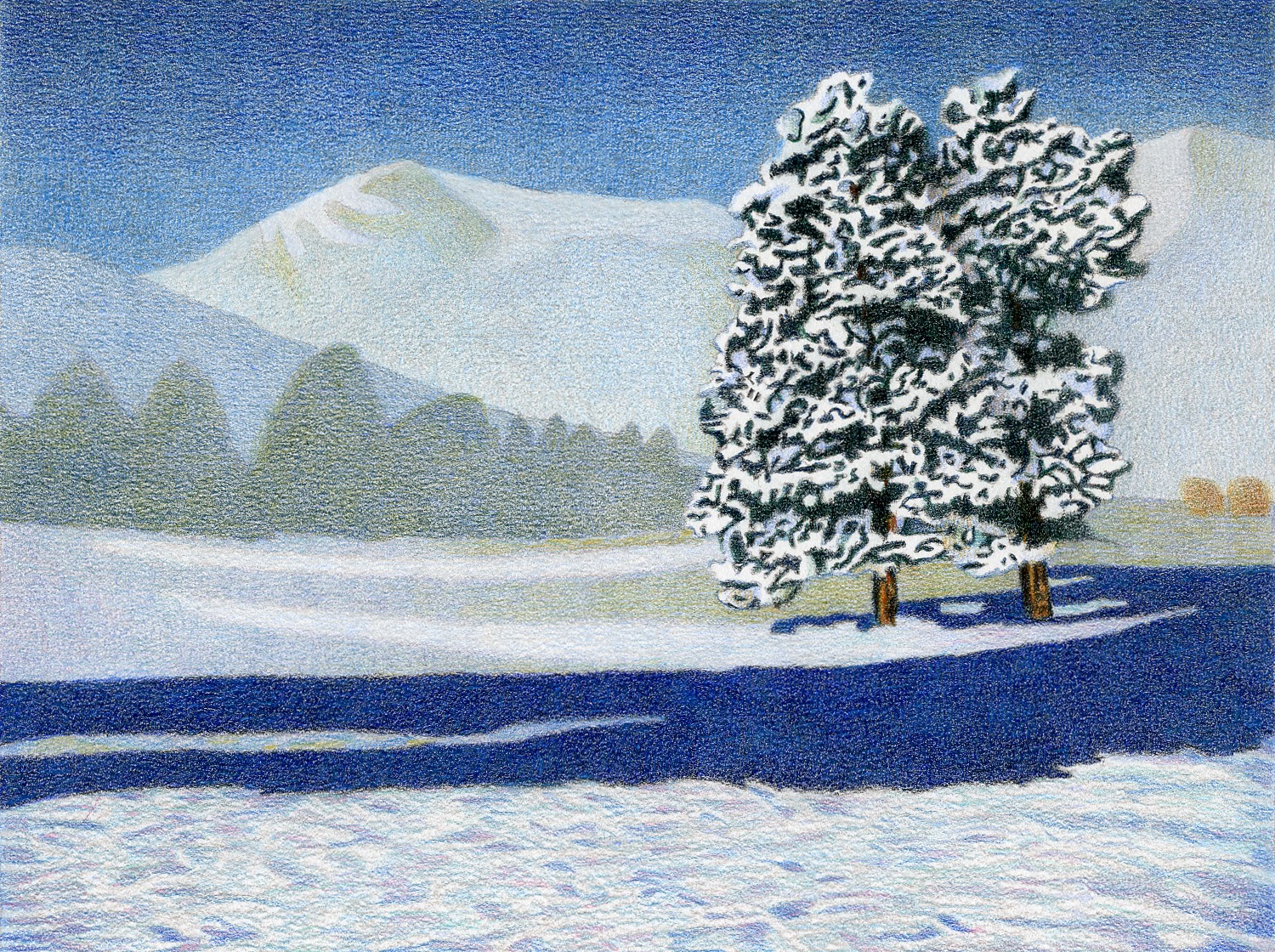In this intricate holiday-themed digital artwork, a beautifully detailed winter landscape is depicted under a vivid, multicolored sky featuring shades of blue, pink, purple, and white. Dominating the central and right side of the image are majestic mountain ranges; the ones on the right are snow-covered, while those to the left are an icy blue. In the foreground, two prominent evergreen trees, heavily laden with snow, stand near the center and right of the image, bordered by a snowy expanse that stretches to the background.

Scattered throughout the scene are patches of snow-covered trees and bushes, creating a dense woodland feel. Adjacent to the evergreens and spreading towards the left, a serene blue body of water adds depth to the scenery. Another smaller area of water is visible at the bottom center of the image, partially covered by a thin ice layer. Horizontally framing the bottom of the picture is a wide strip of snow or ice, signifying the depth of winter's embrace on this picturesque landscape. The complex interplay of colors and elements suggest that this captivating scene is either an exceptionally detailed painting or a high-quality digital creation, evoking the tranquil beauty of a winter wonderland.